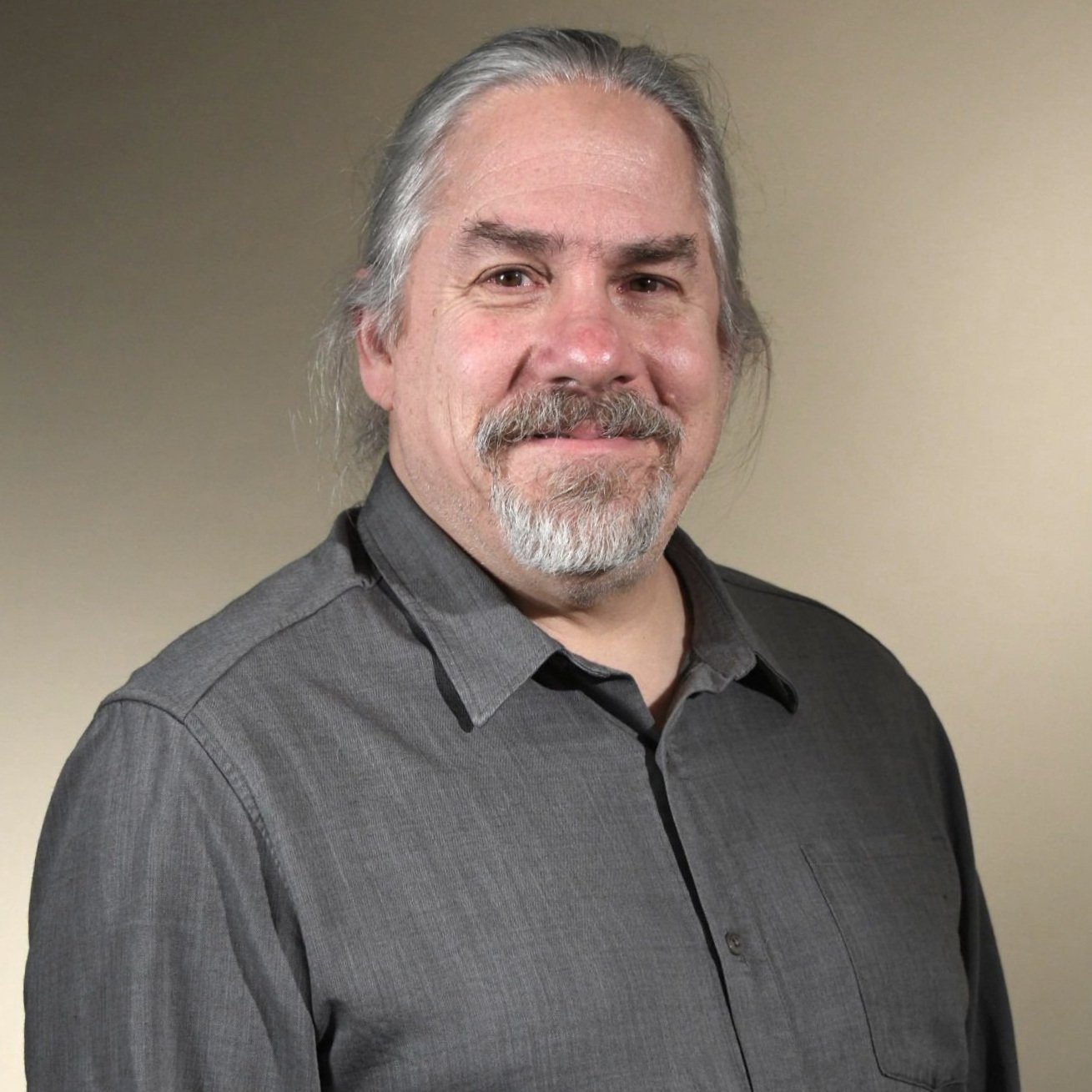The photograph features a middle-aged Caucasian man with pale skin, smiling gently without showing his teeth. His long gray hair is pulled back, and he sports a gray goatee and mustache, as well as black eyebrows and brown eyes. An identifiable wart rests on the right side of his chin. The man, who has a somewhat stocky and portly build, is dressed in a long-sleeve, charcoal gray button-down shirt with a pocket on the left side. The image is cropped at his chest level, with a light brown wall in the background that darkens slightly towards the top left and bottom left corners.